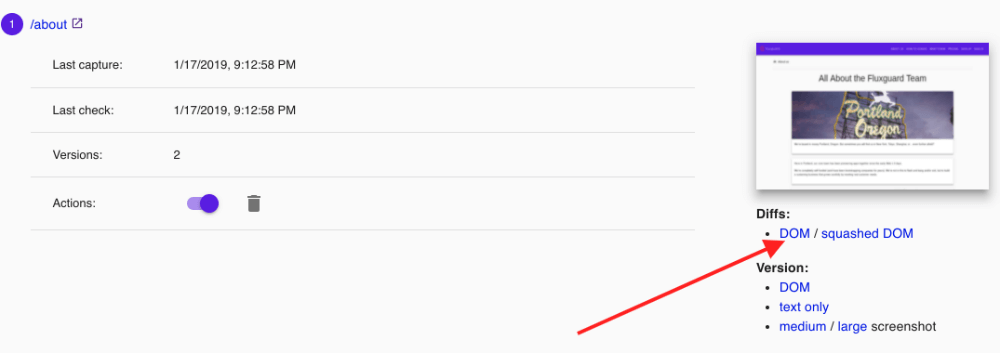This is a screenshot of someone's computer screen with a predominantly grayish background. In the top left corner, there is a purple circle symbol. Adjacent to it is a forward slash followed by the word "about," and next to that is a box resembling a line.

Below this header is a vertical list of four items. The first item is labeled "Last Capture," with the date and time "1-17-2019 at 9:12:58 PM" displayed to its right. The second item states "Last Check," also with the same timestamp "1-17-2019, 9:12:58 PM." The third item reads "Versions: 2," followed by "Actions." The fourth item features a purple "toggle on" button and a trash can icon to the right of it.

On the far right side of the screen, there is a rectangular section with a purple border at the top. This section contains the heading "All About the Flag Guard Team" and a picture captioned "Portland, Oregon" in the middle. Beneath this picture, the word "Diffs" is displayed, followed by several options: "DOM/squash to DOM version," "DOM text only," "Medium/large screenshot." Additionally, a red right arrow originating from the bottom of the screen points upwards toward the section labeled "DOM" listed under the "Diffs" options.